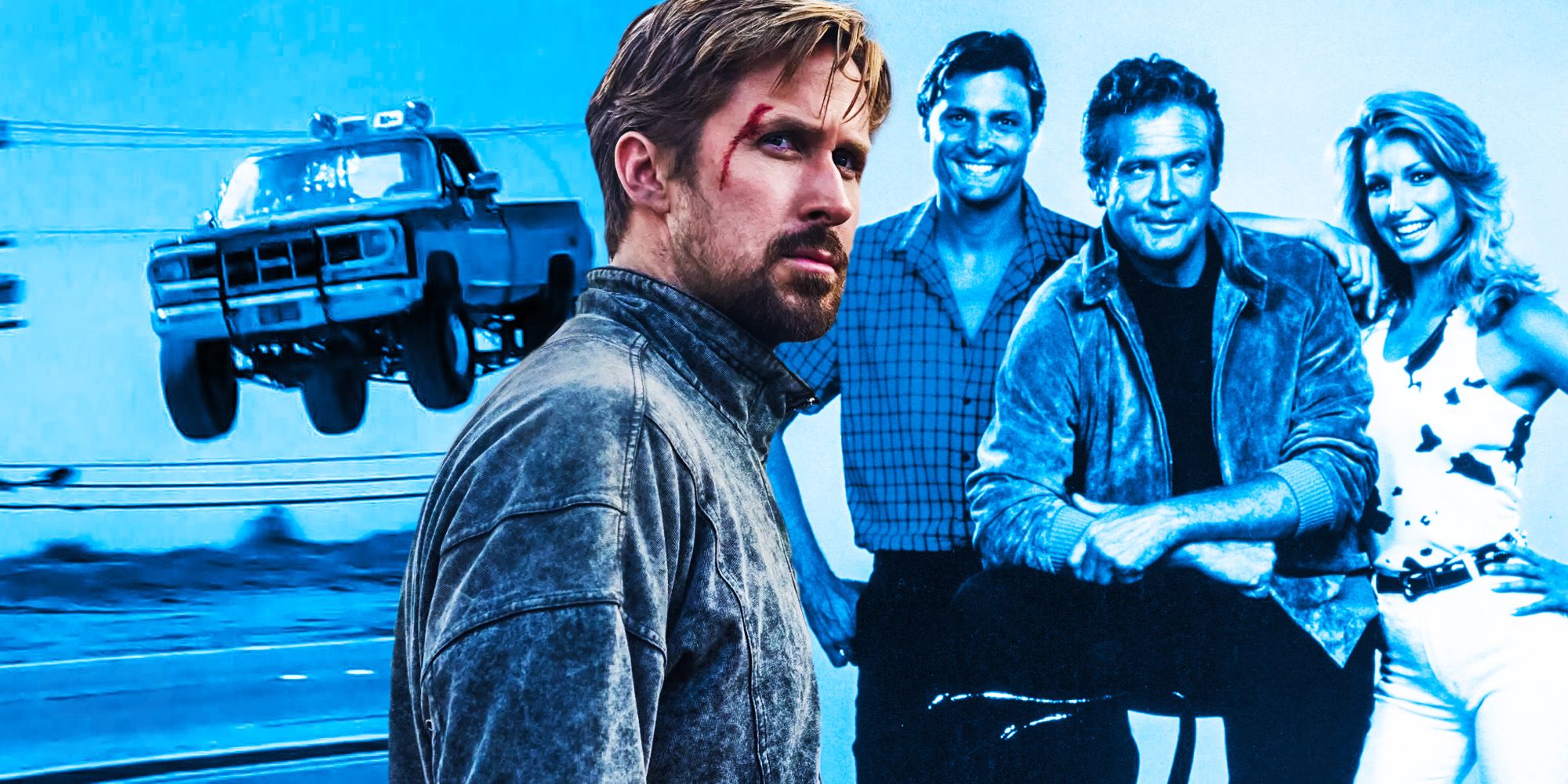This image appears to be a movie poster featuring Ryan Gosling prominently in the foreground. He is dressed in a blue denim jacket, with a small mustache and short beard, bushy eyebrows, and brown hair with highlights. A noticeable cut above his right eye drips blood down his cheek and right elbow, giving him a rugged appearance. He is shown in a side profile, gazing intently into the distance with a stern, distrustful expression.

In the background, the entire scene is bathed in various shades of blue, creating a monochromatic effect. To the left, a large, older model pickup truck, possibly a Ford from the 1980s with floodlights on its roof, is depicted in mid-air as if it has just made a dramatic jump. The truck's position shows it slightly tilted with big tires visible and lit up against the blue horizon lined with trees and telephone wires.

On the right side of the poster, three other characters stand in a group. The central figure, likely Lee Majors, is a white man wearing a blue jacket and dark pants, with one knee propped up on a chair. To his left is another man in a checkered shirt with navy and light blue colors, also probably actors from a different time period. To the right of them stands a smiling blonde woman in a white, possibly tie-dyed tank top and white jeans, completing the trio.

The contrast between Ryan Gosling in natural colors in the foreground and the blue-shaded figures and truck in the background suggests a blend of different eras and styles, possibly indicative of a complex narrative or a crossover theme in the movie.